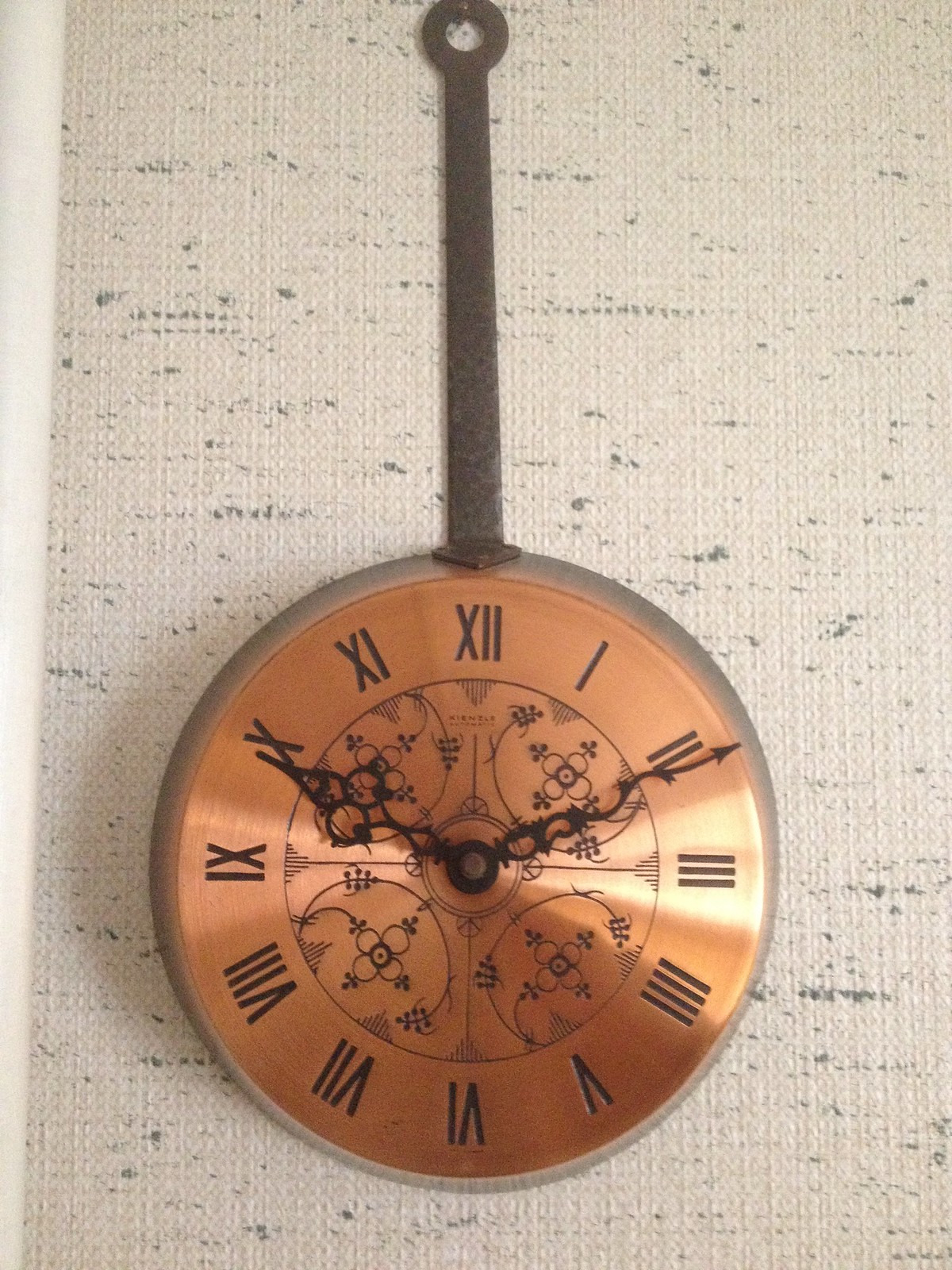This image showcases a vintage-style clock set against a minimalist background. The clock features a circular face with a burnished bronze finish, exuding an antique charm. Roman numerals, such as I for 1 and XII for 12, elegantly mark the hours around the clock's perimeter. Two distinct hands—an hour hand and a minute hand—gracefully point to the time. A sturdy metal rod extends vertically from the top of the clock, culminating in a small, functional loop designed for hanging. The intricate details of the clock, from its metallic sheen to the classic numerals, evoke a timeless, sophisticated aesthetic.